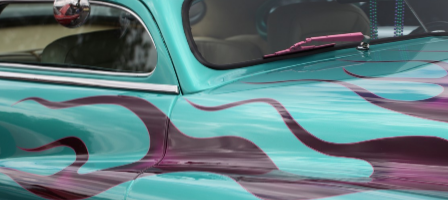This photograph is a small, rectangular image, approximately an inch high and three inches wide. It offers a close-up view of a vehicle's paint job, suggesting it may be a vintage hot rod. The car's main color is a bluish-green, reminiscent of seafoam or light teal, which extends prominently from the right side of the image. 

The vehicle features intricate purple flames that start from the hood and travel down the side, crafting a striking visual contrast. Along the bottom edge of the car, there is an outward-extending fin or fender. The upper left-hand corner of the image reveals a side window with a distinctive round mirror hanging down, possibly silver. Just behind this, a windshield is visible, blending from the center towards the right side of the image, though it is unclear whether it is the front or rear windshield.

Additional details include a light tan interior, barely discernible from the close-up angle. The windshield wipers, noticeable around the front area, appear to be painted in a metal-like burgundy shade that matches elements of the flame design. In the background, an oval-shaped passenger side window trimmed with the same bluish-green color as the rest of the car can be seen, further adding to the vehicle's unique aesthetic.